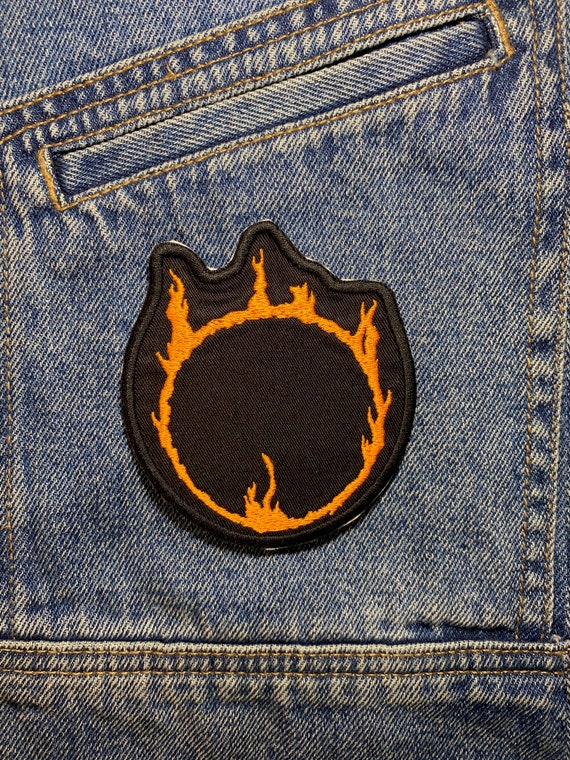This close-up color photograph in portrait orientation captures the intricate details of a portion of stonewashed blue denim, specifically a section of a pair of jeans featuring a unique patch. The focus of the image is a diagonal slash pocket, accentuated by bold yellow-golden stitching, which rests near the upper-left portion of the photograph. Just below this pocket is a distinctly striking patch, centrally positioned within the frame.

The patch itself is predominantly black, with an irregular shape that is circular along the bottom but more jagged along the top edges, adapting to the fiery design it portrays. A meticulously stitched orange ring of fire forms the core of this patch, with flame peaks shooting out variably in different directions—most notably from the bottom, the right side, and the top. The background of the patch and its edging are defined by black stitching, with heightened edges outlining the more prominent flames, giving it a dynamic, three-dimensional appearance.

Running along the edge of the image, the seams of the denim trace a path across the bottom, then upwards along the right side before descending back toward the left, just skirting the edge of the patch and the pocket. The photograph embodies a realist style, capturing the texture and composition of the denim material and the detailed craftsmanship of the patchwork.